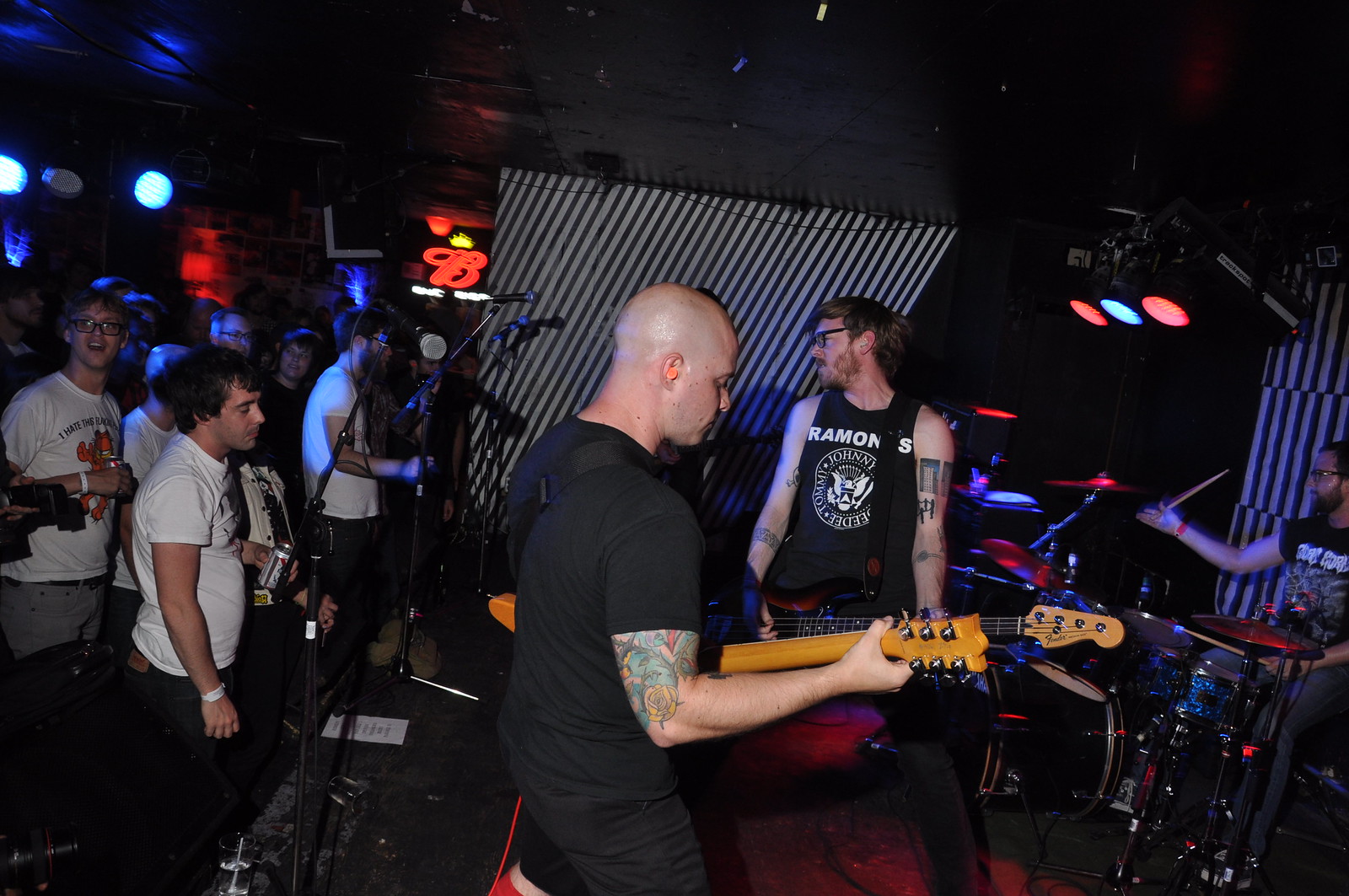This photograph captures the energetic atmosphere of a rock concert taking place in a bar or nightclub. On the stage, three musicians are engaged in a high-energy performance. On the right side of the image, a guitarist is seen with his back turned to the crowd, standing next to another guitarist who is more centrally positioned and wearing a black Ramones t-shirt. The second guitarist, recognized by his glasses and scruffy beard, has his legs spread out and turns his head towards the audience. In the background, the drummer is captured in action, poised to strike the cymbals or chimes with a drumstick raised in the air. He is also dressed in a black t-shirt, possibly featuring another band. The lighting above them casts red and green hues, adding to the vibrant scene. In the foreground on the left, a crowd of mostly men in white t-shirts, alongside others in black, watches the band while holding beers. A Budweiser sign is part of the décor, affirming the bar setting. The dark walls and stage positioning central in the image contribute to the intimate, club-like atmosphere of the concert.